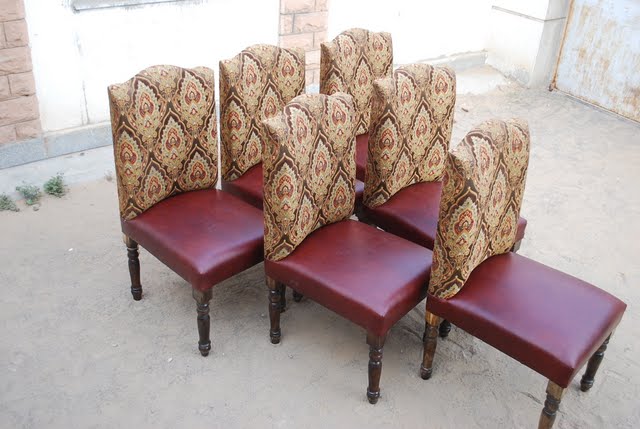In the image, six intricately designed chairs are arranged in a formation resembling bowling pins, with the front chair positioned in the bottom right corner and the others extending diagonally upwards to the left. Each chair features a seat covered in burgundy leather and has decorative backs with intricate designs reminiscent of Hindu or Middle Eastern art, displaying mandala or fractal-like patterns in varying shades of dark or light brown to greenish tones. The legs of the chairs are crafted with lathe-turned ornamentations. The setting appears to be an empty room or warehouse with worn white walls, sunlight streaming in through open windows, and a brick wall visible in the top left. The scene is brightly lit, suggesting an outdoor yet enclosed environment.